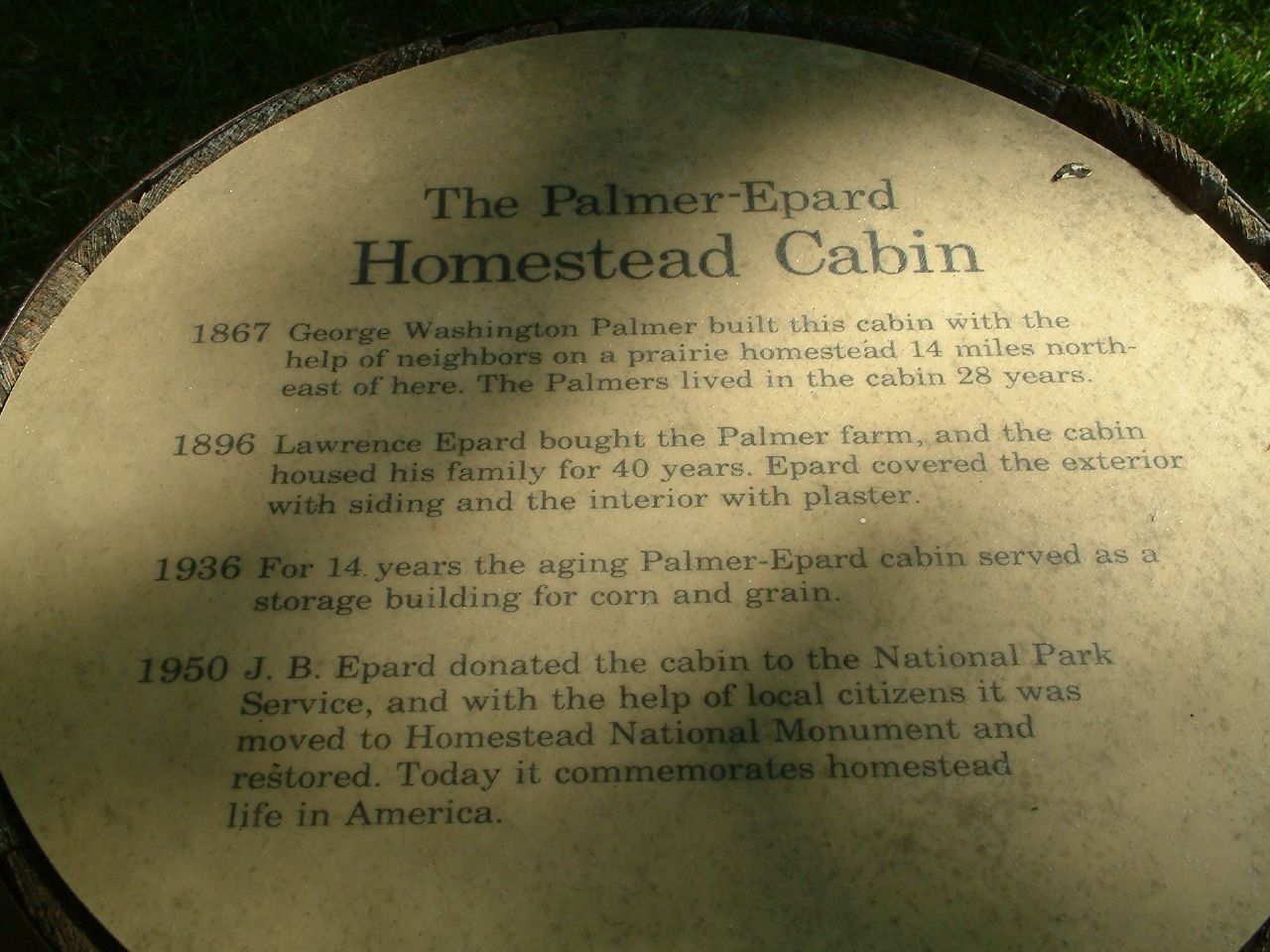The image depicts a round commemorative plaque with a wooden border, set on the ground with patches of grass visible in the upper right and left corners. The plaque is titled "The Palmer-Eppard Homestead Cabin" and chronicles the history of the historic cabin. It reads:

"1867: George Washington Palmer built this cabin with the help of neighbors on a prairie homestead 14 miles northeast of here. The Palmers lived in the cabin for 28 years.
1896: Lawrence Eppard bought the Palmer farm, and the cabin housed his family for 40 years. Eppard covered the exterior with siding and the interior with plaster.
1936: For 14 years, the aging Palmer-Eppard Cabin served as a storage building for corn and grain.
1950: J.B. Eppard donated the cabin to the National Park Service. With the help of local citizens, it was moved to the Homestead National Monument and restored. Today, it commemorates homestead life in America."

The plaque is situated outdoors, where the play of light and shadows adds depth to its appearance, indicating the passage of time and the rich history encapsulated in this homestead cabin.